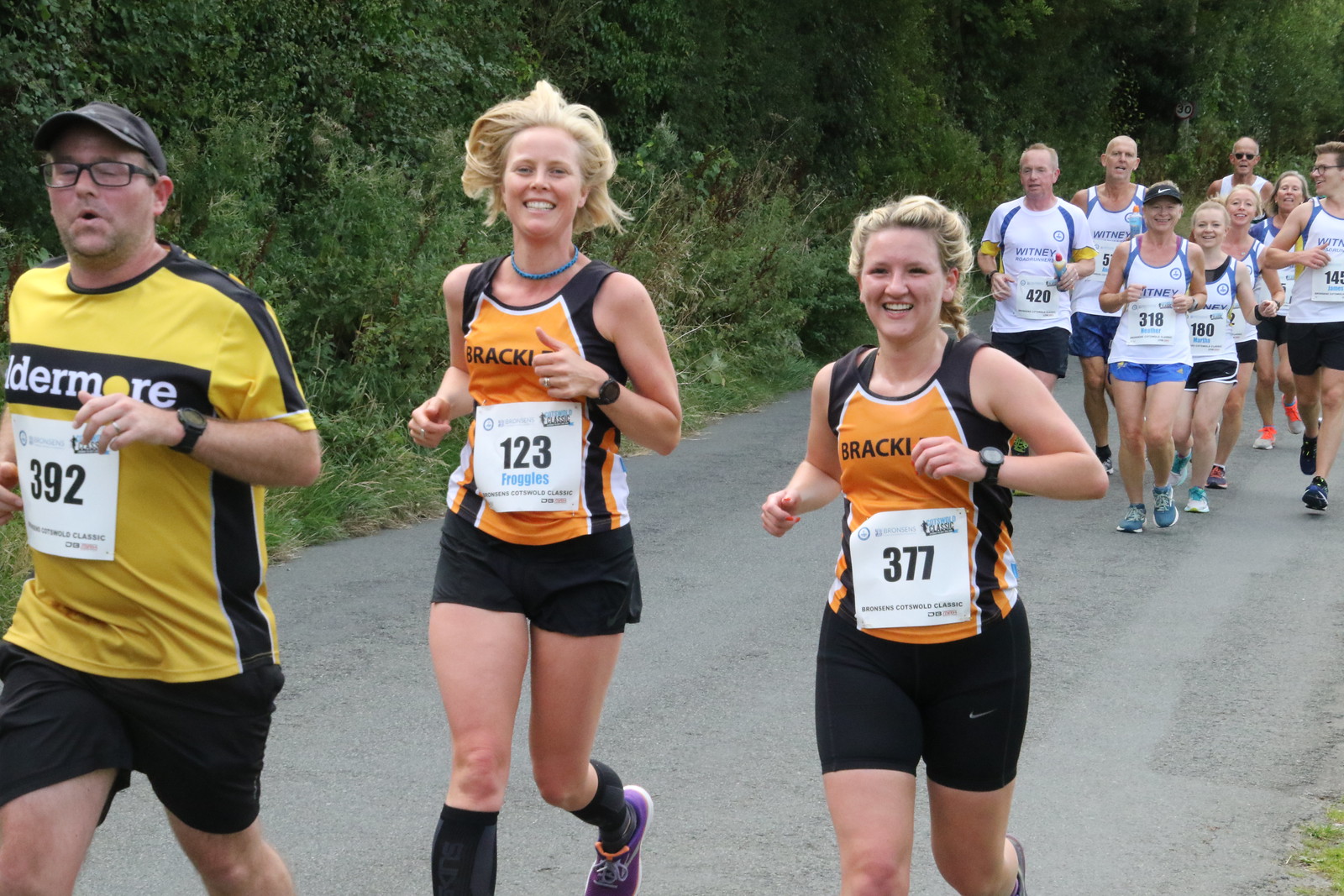The image captures a marathon scene on a Blacktop Road lined with greenery, featuring a diverse group of runners of varying ages. Prominently in the foreground, there is an older man wearing a yellow shirt with the number 392, a grey cap, and grey-frame glasses. Close behind him is a fit woman sporting an orange tank top that says "Froggies" with the number 123. She has lean, muscular legs and is blonde. To her right is another blonde woman, slightly shorter and fuller-figured, also wearing an orange and black jersey, numbered 377, with blonde braids and black shorts. She is smiling towards the camera. In the background, a crowd of runners can be seen, all donning white outfits that read "Whitney Road Runners," featuring various numbers such as 420, 318, 180, and 145. The marathon is part of the Scottswold Classic and Bronson's Cotswold Classic events.